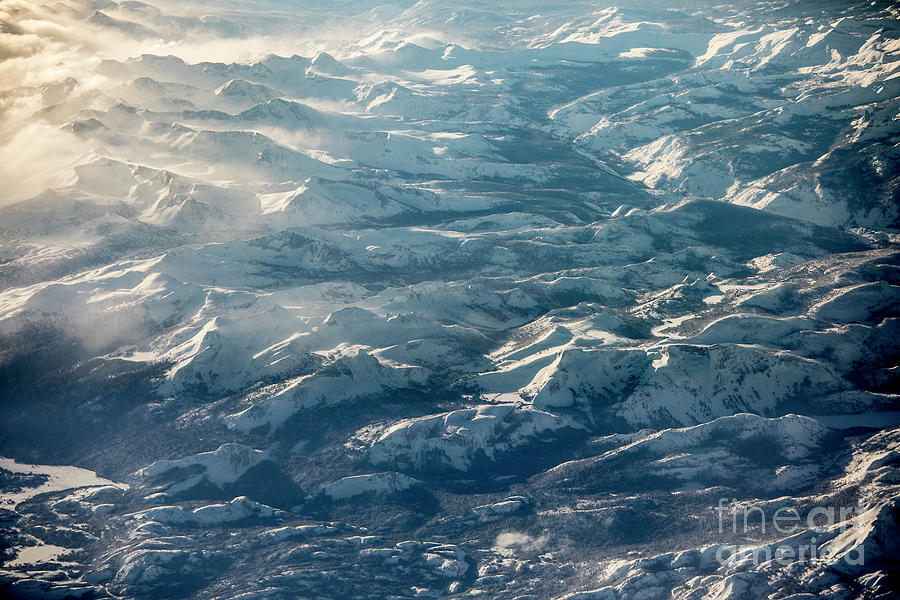An aerial photograph captures a breathtaking, snow-covered mountainous landscape, showcasing various rising levels of rugged terrain laid next to each other. The perspective, possibly taken from a helicopter or drone, reveals both jagged and rolling peaks, with mist or fog settling into the valleys, creating an ethereal atmosphere. The mountains, with their dark ridges contrasting sharply against the snow, stretch across the scene, which is illuminated by a strong light source coming from the top left, casting dynamic shadows and highlights. The bottom left corner hints at either a river, melting snow, or a small puddle, adding a subtle touch to the composition. In the bottom right corner, the words "Fine Art America" appear in transparent white font, indicating that this stunning photograph is a piece of artwork available for sale.